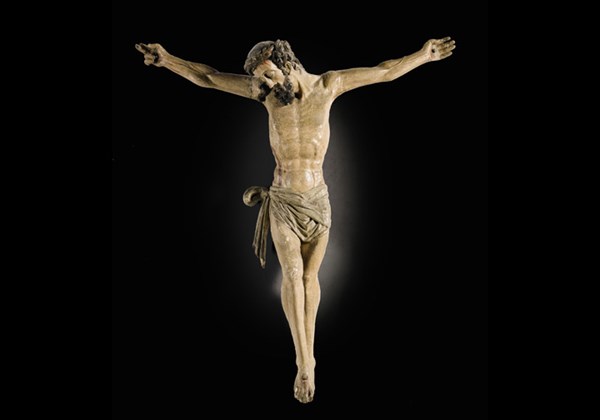The image depicts a highly detailed and emotive statue of Jesus Christ in a crucifixion pose against a stark black background. The statue appears to be made from white stone or wood, with attention to fine details such as a grayish tint in the curly hair and a short beard. The figure is shown emaciated, with visible ribs and a solemn expression. His head is drooped down to the right side, eyes closed, with streaks of blood on his forehead suggesting a crown of thorns. Both arms are outstretched horizontally, with nails driven through the palms. He wears a light brown loincloth, tied on the left side, covering his pelvic area. His legs are crossed at the ankles, with one foot on top of the other, fixed together by a single nail. Adding a divine touch, there is a subtle white glow around the midsection of his body, contributing to the spiritual and somber atmosphere of the scene.